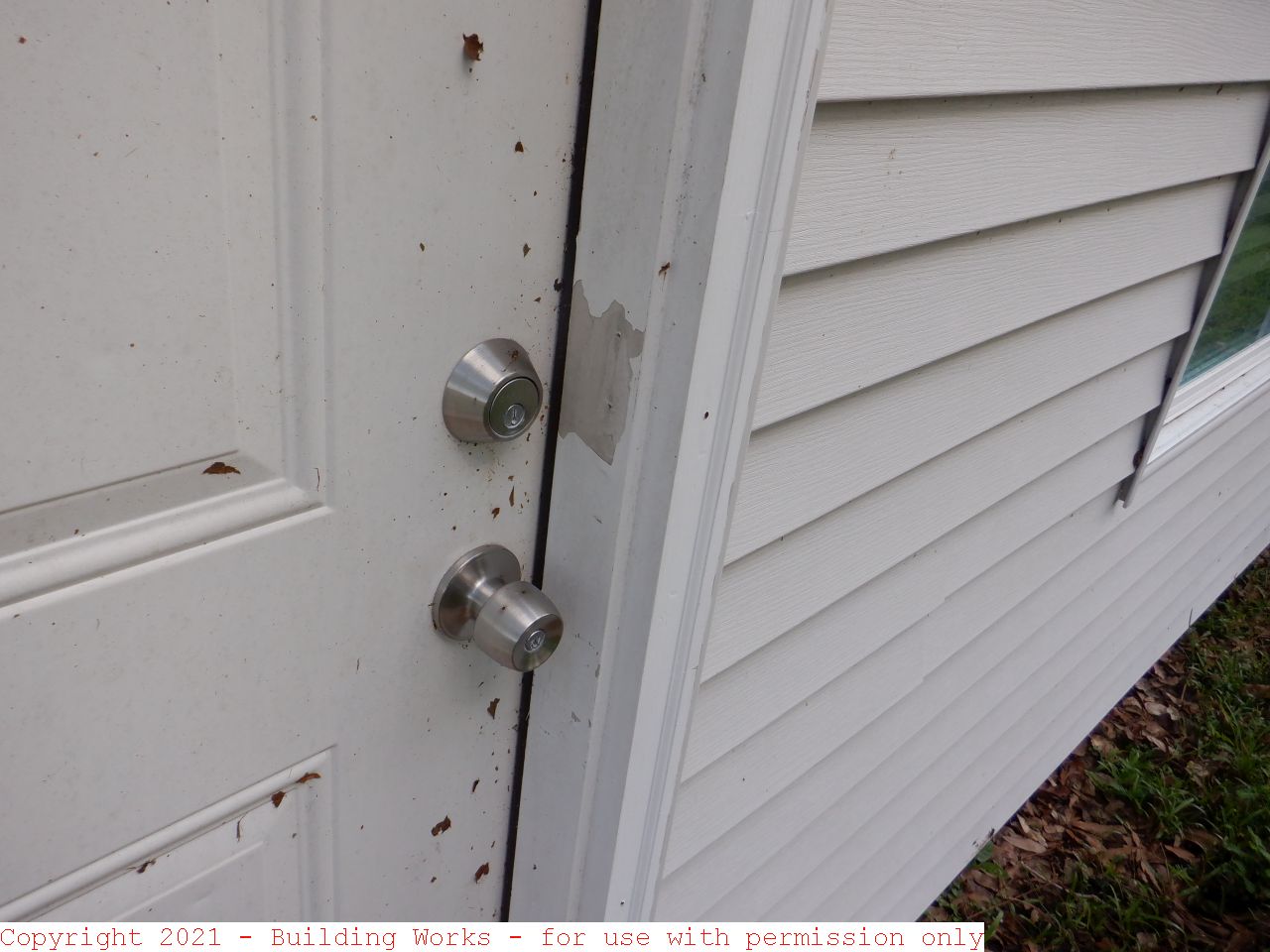This outdoor photograph captures a close-up, angled view of a dingy, white front door on the left side of the frame. The door features a round, silver doorknob and a matching deadbolt. The white paint on the door and the surrounding frame is visibly chipped, particularly around the deadbolt, revealing a gray color underneath. Brown specks and dry leaves clutter the handle's side edge of the door, adding to its weathered appearance. The house's white paneled siding extends to the right side of the image, where a partially visible window is framed in silver. The lower right-hand corner shows a patch of green grass mixed with dirt and brown leaves. In the bottom left corner, there is a white rectangle with red text that reads: "copyright 2021 building works for use with permission only." The image is taken during the day.